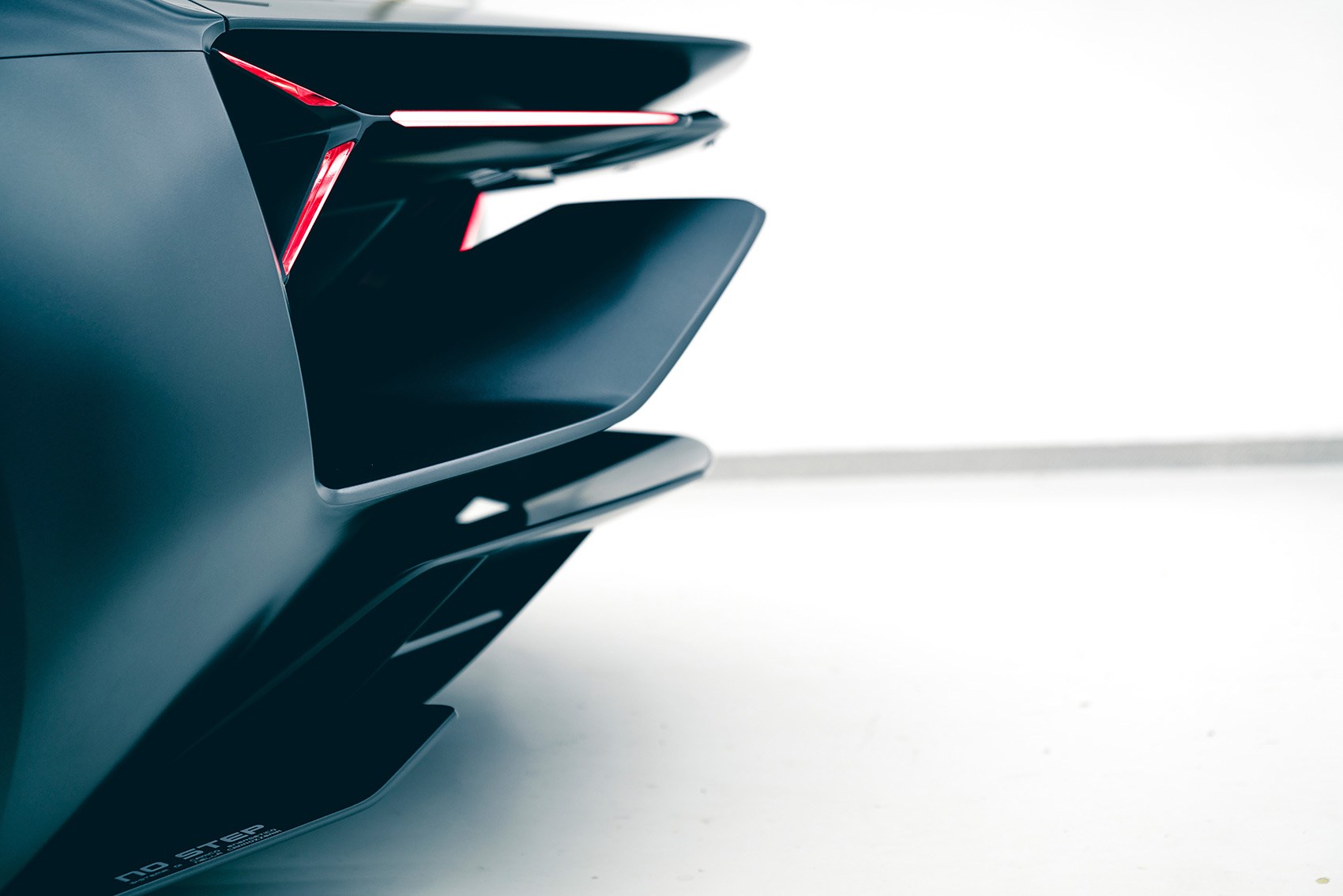The image depicts the back of a futuristic, high-tech sports car or possibly a concept vehicle with a grayish-black metallic finish. The structure includes what might be parking lights or turn lights, positioned near an intricately designed exhaust-like area close to where the trunk would typically be. This section slopes down at a lower angle, contributing to its sleek appearance. Notable features include red elements and a "No Step" label on a small protruding platform, hinting at aviation-inspired design cues. The abstract, space-age aesthetic suggests it could also belong to a high-tech concept motorcycle or even a piece of advanced machinery, emphasizing its modern and otherworldly vibe.